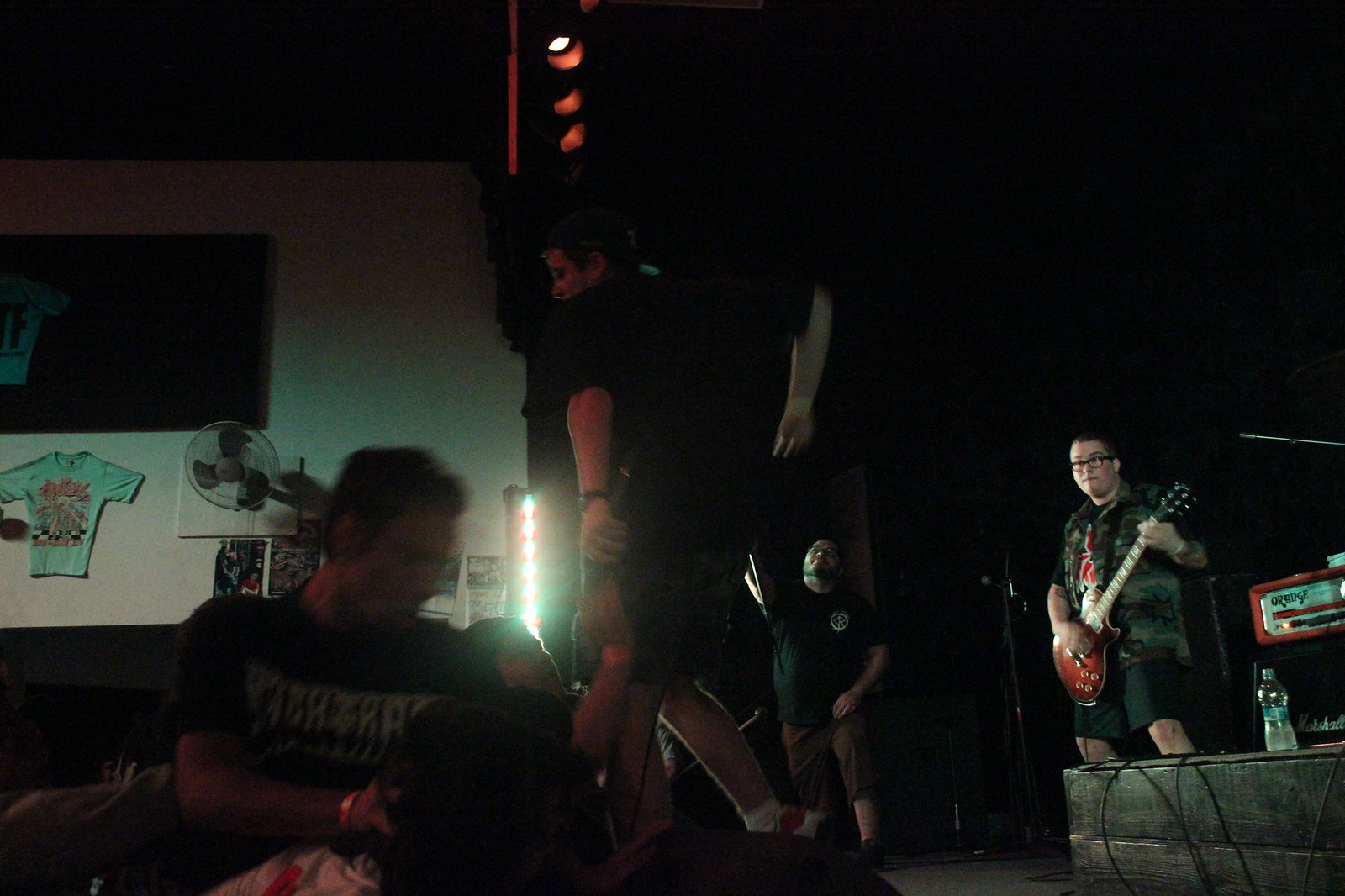In this color photograph, a rock band is captured during a live performance, likely in a dimly lit club or bar. Three band members are on stage, predominantly dressed in black. On the right, a young man plays an electric guitar, smiling as he glances toward the center of the stage. Near him, an orange amplifier is visible. In the middle of the stage, another band member, clad in a black t-shirt and camo shorts, is supported, possibly pushed, by a fan from the audience who is at the very edge of the stage. The interaction suggests an autograph or handshake. The left side of the stage features a third band member in a more distant position, though blurriness makes details hard to discern. The setting includes hanging posters, fans, and a t-shirt displayed on a white cardboard, hinting at a classic rock concert atmosphere. Motion blur throughout the photo suggests dynamic movement, as the photographer captured the energetic scene from up close.